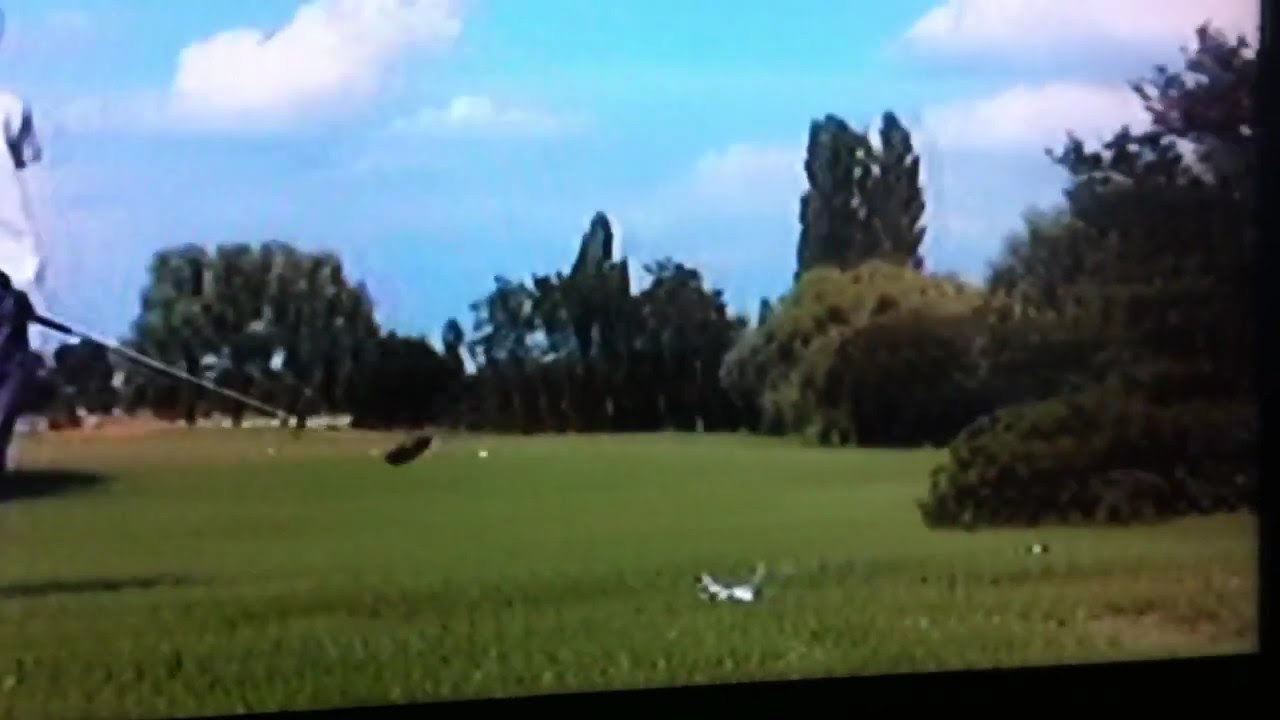This image, likely a still from an old VHS tape or a photograph of a TV screen, depicts a scene on a golf course during a mostly sunny day. The overall quality is very pixelated and the shot appears out of focus, with a black border on the right side and lower right side of the rectangular frame. Dominated by vibrant green grass and tall, lush trees in the background, the scene also includes a bright blue sky with scattered white clouds. Positioned on the far left of the image is a golfer dressed in dark pants and a white shirt, holding a wooden golf club parallel to the ground, amidst a swing or just after swinging. Towards the lower center of the image is a small white object, which is indistinct but hints at being some sort of debris. This detailed landscape captures both the clarity and vibrancy of the outdoor setting as conveyed through the flawed medium.